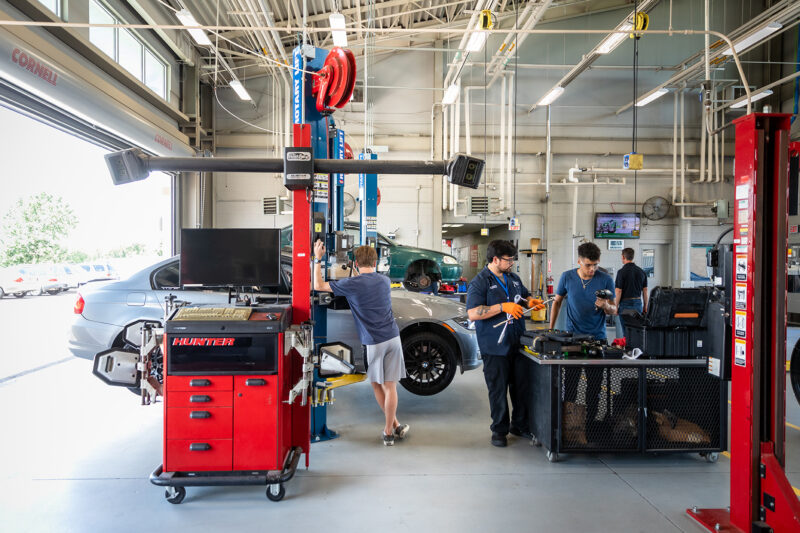The photograph depicts a spacious, well-lit auto repair shop with tall ceilings and multiple service bays. The shop features modern equipment, including red lifts and tool cases from the company Hunter. Two cars are elevated on the lifts; one is slightly obscured by equipment, while the other is fully visible in the background. The shop has a large door on one side that is open, revealing a parking lot outside. Inside, four men are engaged in various tasks: two technicians are working with tools, while another man, possibly a customer, stands in gray shorts, a blue shirt, and sneakers, leaning against a computer monitor and observing his car. The men are wearing dark-colored clothing. The floor is clean, gray concrete, and the shop is illuminated by both natural light and numerous fluorescent lights overhead. In the background, several drop-down electrical lines and light-colored walls enhance the modern and organized appearance of the garage. There's also a hint of a waiting room with a television located at the back-right side of the shop.